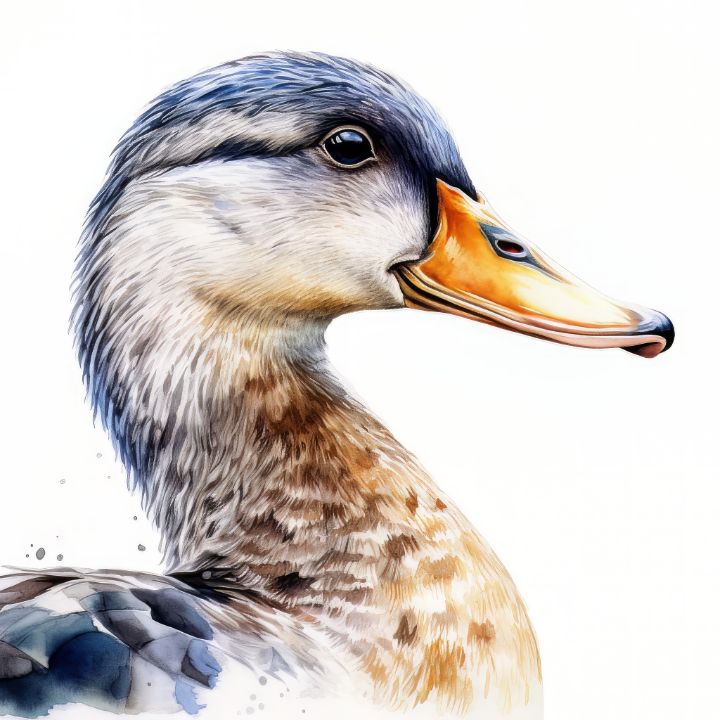This is a detailed, realistic watercolor painting of a duck set against a white background. The painting features only the upper part of the duck's body, capturing its head, neck, and a portion of its back in exquisite detail. The artist has employed a minimalist palette consisting primarily of raw umber and yellow ochre, using a combination of dry and wet brush techniques. This creates a vivid, lifelike texture that almost allows you to feel the feathers. The duck's plumage showcases a harmonious blend of black, white, and various shades of brown, including spots of tan. Its orange bill transitions into a tannish color with a black tip, while the eye is black-ish brown, encircled by a dark band extending over the head. Flecks of paint are strategically placed to emphasize the hand-crafted nature of the artwork. The layered colors and precise brush strokes contribute to a strikingly realistic and tactile impression of the duck's feathers.